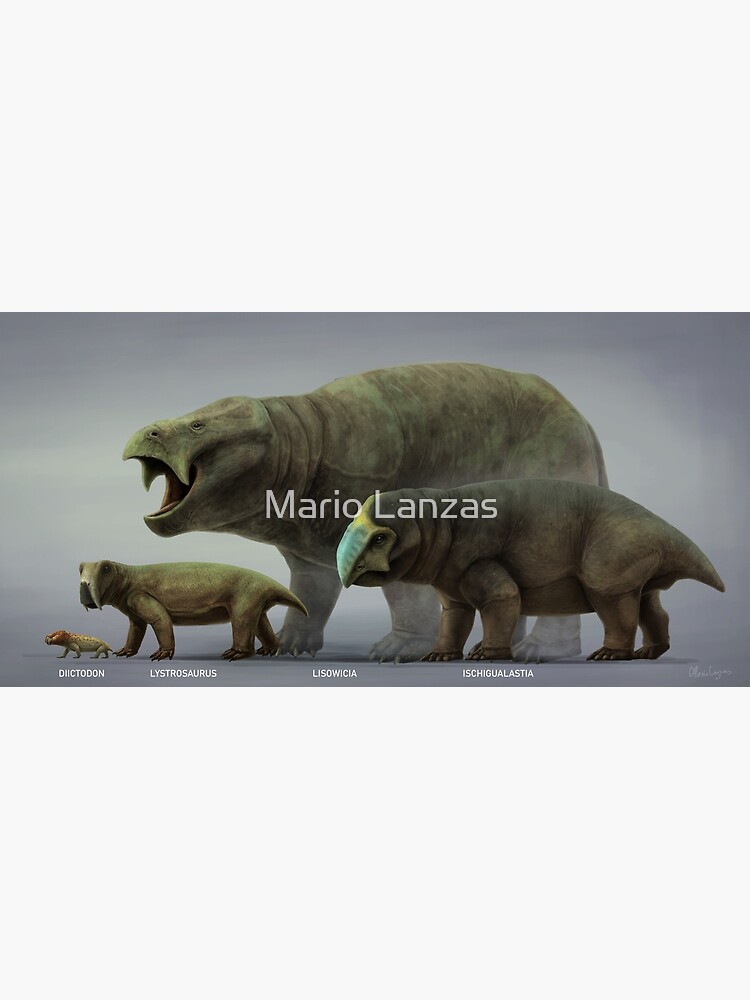The illustration depicts a series of four prehistoric creatures rendered in what appears to be a 3D style. The background is a uniform, bleak grey that highlights the stark figures of the creatures. Starting from the left, the smallest creature, labeled Dictodon, resembles a lizard with greenish skin and mild yellow and grey elements. To its right is a significantly larger Lystrosaurus, approximately eight times the size of the Dictodon. The largest creature, Lysowikea, dominates the center of the image, towering over the others and standing out with its immense size, possibly twice as large as the Lystrosaurus. On the far right is the medium-sized Ishigualastia, characterized by its beak-like features. The creatures, presented in a progression of sizes and distinct morphology, appear almost mythical, yet indicative of actual prehistoric entities that have either evolved or become extinct.